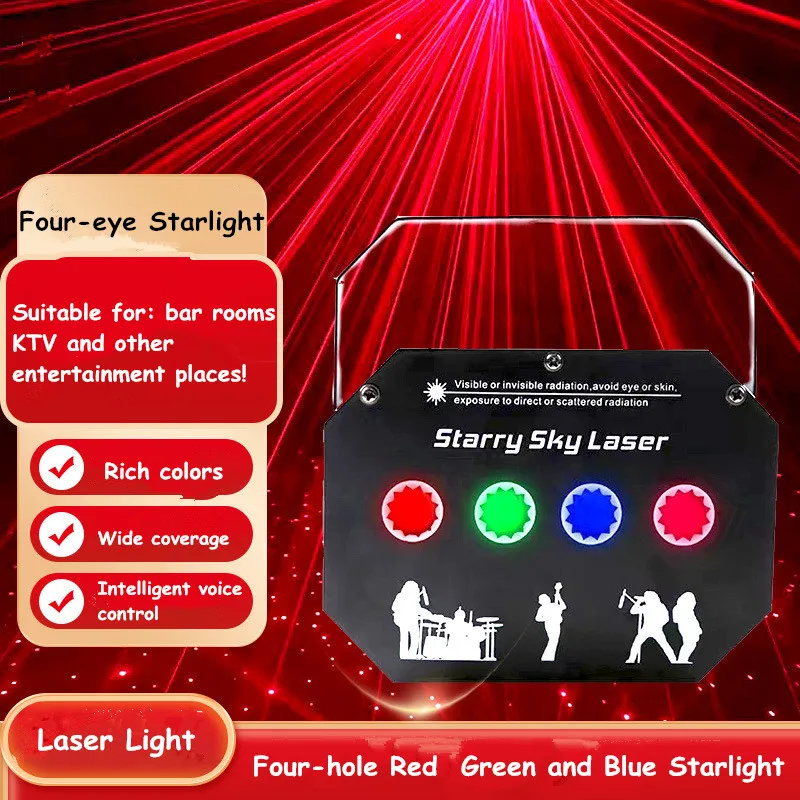This image showcases an infographic for a "Starry Sky Laser" on an eye-catching, radiant red background that resembles red rays converging towards filaments, reminiscent of optic fiber formations. The bold red background contrasts with the white filaments, creating an almost stellar effect. Centered prominently, "Laser Light" is displayed in a white Comic Sans Serif font, creating a three-dimensional and shiny appearance. It elaborates on the "Four Hole Red, Green, and Blue Starlight" features. 

Above this, there is a black metal plate-like image with a handle, displaying the text "Starry Sky Laser" in white font, warning "Visible or Invisible Radiation: Avoid Eye or Skin Exposure to Direct or Scattered Radiation." This area also showcases four laser colors: dark red, green, blue, and a lighter magenta. Below, the silhouettes of a rock band are depicted in white against a black background, featuring musicians playing drums, guitar, and singing.

On the left margin, taking up most space, it states "4i Starlight" on a beige background, and specifies the product is "Suitable for Bar Rooms, KTV, and Other Entertainment Places." Three red buttons with checkmarks highlight features: rich colors, wide coverage, and intelligent voice control. This detailed infographic effectively combines vivid visuals and clear textual information, portraying the broad capabilities and applications of the laser light product.